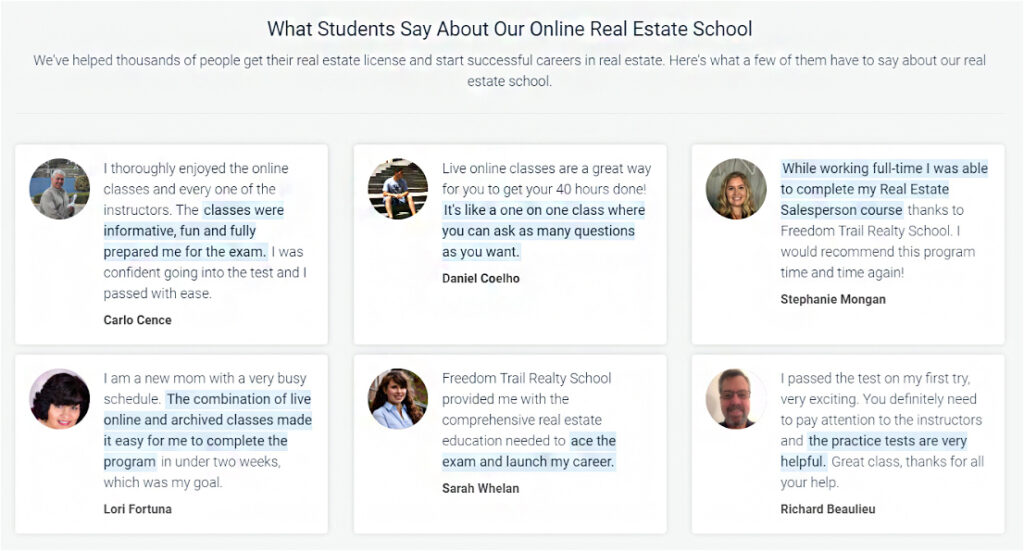The image features a light gray background with a header at the top that reads, "What students say about our online real estate school." The caption explains that the school has assisted thousands of individuals in obtaining their real estate licenses and launching successful careers in real estate. 

Below the header, there are six white squares, each containing a round profile picture of a testimonial provider and their corresponding comment. 

1. The top left square features a testimonial by Carol Kamps, stating: "I thoroughly enjoyed the online classes and every one of the instructors. The classes were informative, fun, and fully prepared me for the exam. I was confident going into the test and I passed with ease."

2. Directly beneath Carol's comment, Lori Fortuna shares her experience: "I'm a new mom with a very busy schedule. The combination of live online and archive classes made it easy for me to complete the program in under two weeks, which was my goal."

3. In the top middle square, Daniel Coelho comments: "Live online classes are a great way for you to get your 40 hours done. It's like a one-on-one class where you can ask as many questions as you want."

These testimonials collectively highlight the flexibility, quality, and effectiveness of the online real estate school’s program.